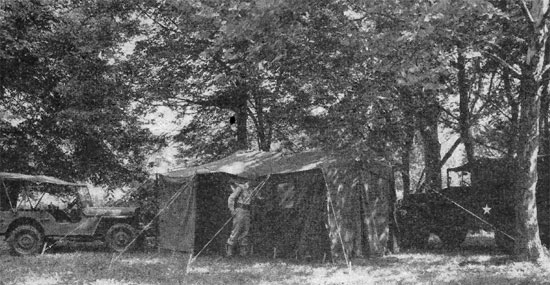In this historic black-and-white photograph, we're looking at what seems to be a military camp set amidst a grove of tall, lush deciduous trees. Dominating the scene is a large square military-style tent, likely a six or eight-man tent, equipped with a window. To the left of the tent is a green open-air jeep with a fabric canopy, and to the right, a darker military jeep with a star emblem on the driver's side door, suggesting it might be a troop transport vehicle. Standing in front of the tent is a figure, possibly a soldier in uniform with a thick black belt and carrying a backpack. The figure's posture is somewhat unnatural, leaning forward, which might indicate age or damage to the photograph, making the details grainy and less discernible. The lighting suggests it's daytime, with sunlight filtering through the treetops, illuminating a small patch of grass in the foreground.